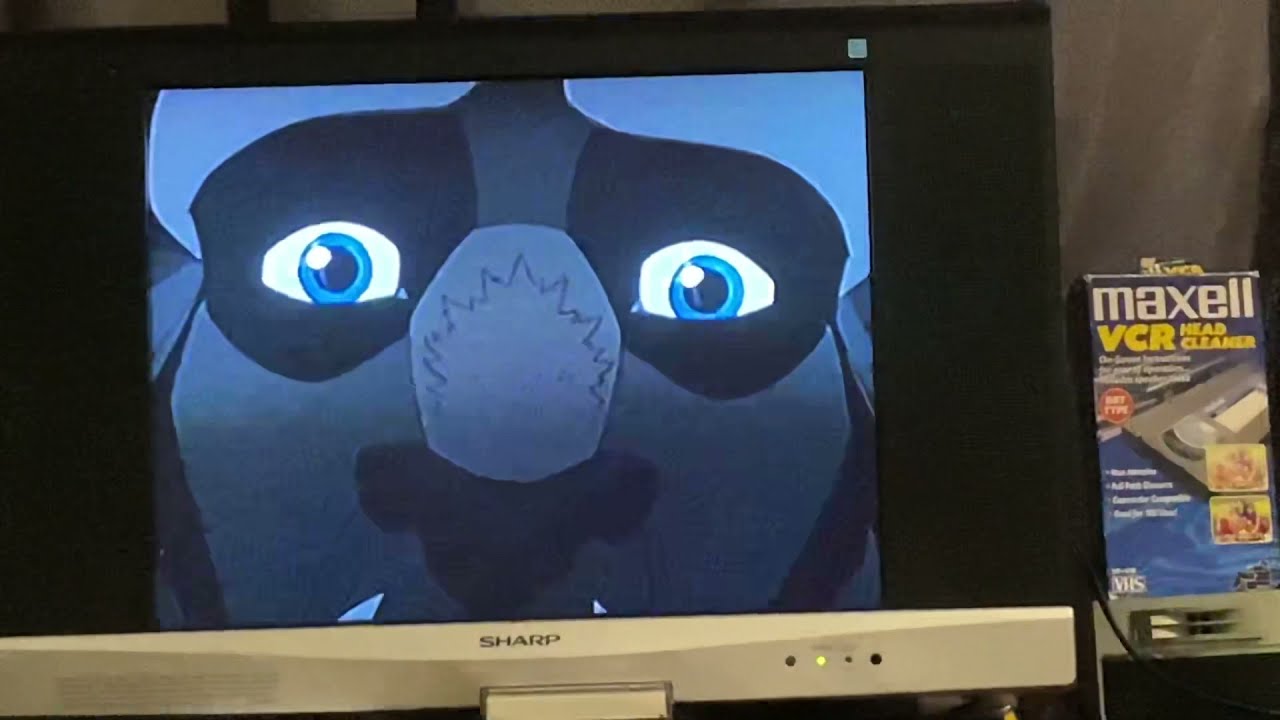The image depicts a Sharp television displaying a close-up of an animated character's face, prominently featuring a large blue face with a gigantic nose, potential fangs, and big white eyes with blue pupils. This expressive character might be from a cartoon or video game, potentially resembling Beast from Beauty and the Beast. The TV has a black screen encased in a silver base where the buttons and lights are located, suggesting it is an older tube model, likely from the 90s. To the right of the TV, there's a Maxell VCR Head Cleaner box, which includes an image of a VHS tape and is partially obscured text. The colors in the scene include blue, light blue, black, beige, white, gray, yellow, and red, all inside a horizontal rectangular frame. The setting seems to be indoors.